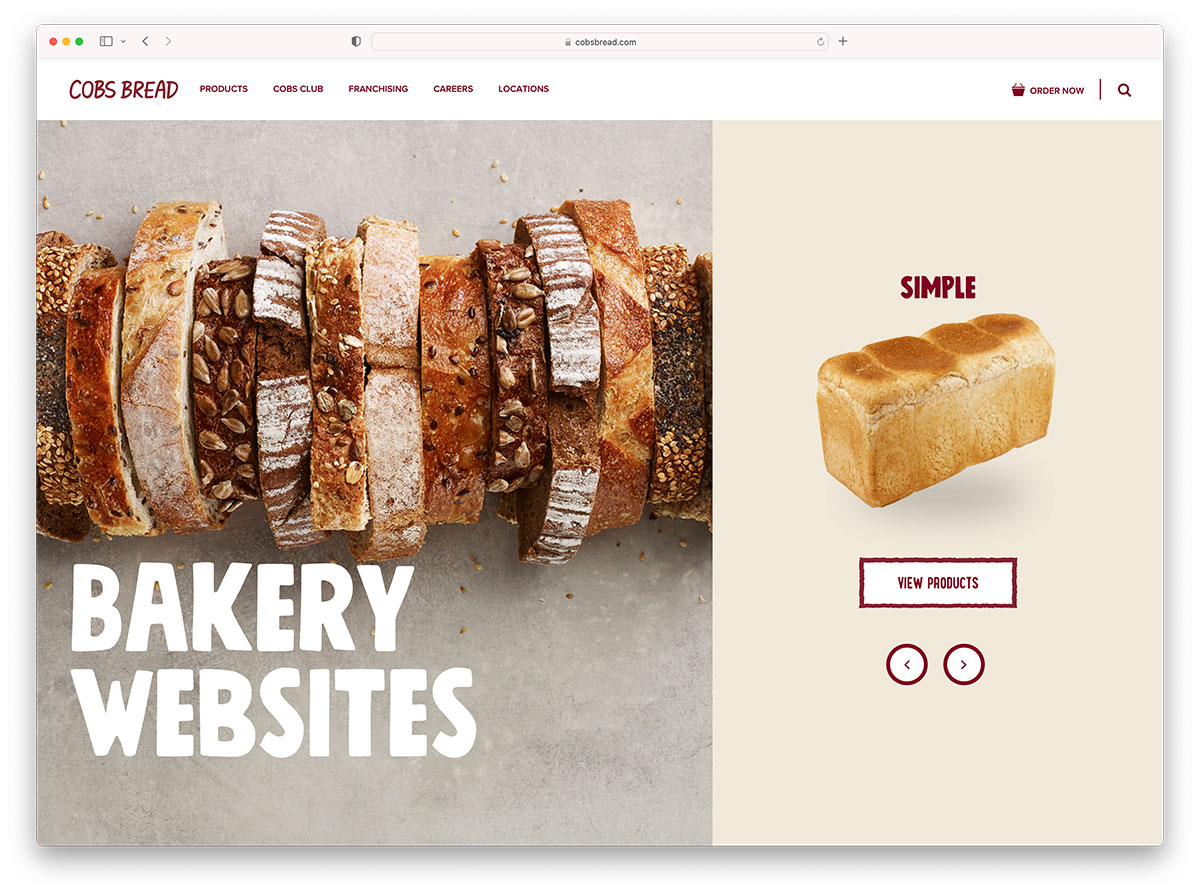The image is a screenshot of the homepage for a bakery website called "Cobs Bread" (spelled C-O-B-S). The top of the website features the name "Cobs Bread" accompanied by colorful icons: red, yellow, and green. Just below, there are navigation options labeled Cobs Bread Products, Cobs Club, Franchising, Careers, and Locations.

On the left side of the page, there's a photograph of various slices of bread, each representing different types of bread, some with nuts and others in varying shades from white to dark brown. Overlaid on this image, the text "Bakery Websites" is prominently displayed in white.

On the right side, there's a full loaf of white bread set against a tan background. Above this loaf, the word "Simple" is written in red text. Below the loaf, there’s a white box encircled by a red outline, featuring the text "View Products" with arrows for navigation beneath it. The overall color palette of the website includes beige, tan, brown, white, and chocolate hues.